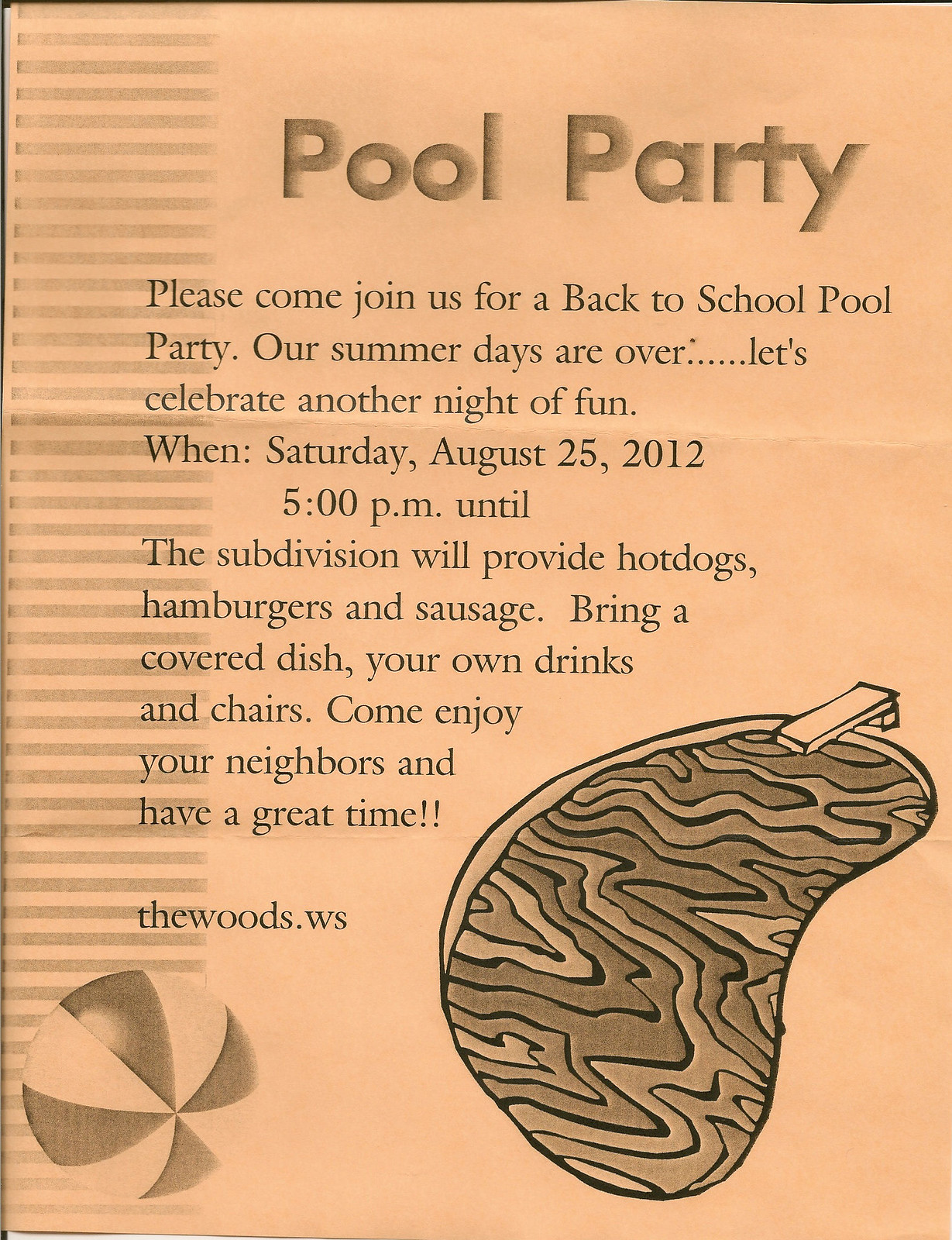The invitation shown here is a scanned copy of a back-to-school pool party invite. Printed on a peach-colored paper, possibly faded due to sunlight, it has a noticeable crease across the top half suggesting it was folded at some point. At the top, in large bold font, it reads "Pool Party." Below this, in standard black lettering, it invites guests: "Please come join us for a back-to-school pool party. Our summer days are over. Let's celebrate another night of fun. When? Saturday, August 25, 2012, 5 p.m. until..." No end time is specified, just that the subdivision will provide hot dogs, hamburgers, and sausage. Attendees are asked to bring a covered dish, their own drinks, and chairs. "Come enjoy your neighbors, and have a great time," it encourages, and it concludes with "TheWoods.ws."

The invite is visually accented with a clipart-style image of a pool with a diving board in the lower right corner, where waves and ripples in the water can be seen. In the lower left corner, there's a colorful image of a beach ball with white and colored stripes. Additionally, the paper features different shaded stripes along the left side, adding to the summery theme. All the text is centrally aligned and typed in a standard black font.